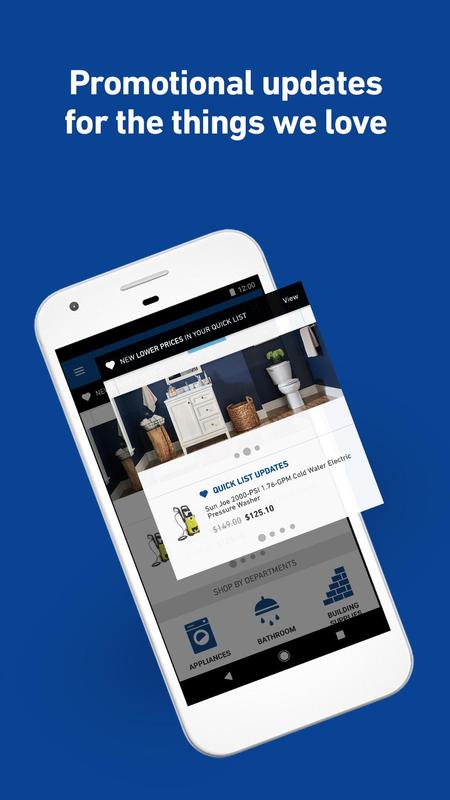In this image with a dark blue background, there is centered text at the top featuring two lines in large, bold, white font that read, "Promotional updates for the things we love." At the bottom of the image, a smartphone is displayed, tilted slightly to the left with its top pointing around the 11 o'clock position. The phone has a white bezel around its perimeter. 

The smartphone's screen showcases what appears to be a business’s sales page focusing on quick list updates. A notable feature on the screen is a section that has been highlighted and elevated slightly to the right, creating a 3D effect. The top of this highlighted section contains a black banner with a heart icon, accompanied by the text, "New lower prices in your quick list," and a "View" button on the right. 

Beneath this banner, the background is white, displaying an image that resembles a residential bathroom setting. Below this, navigational dots indicate the presence of additional content; the central dot is prominently bold, suggesting it is the current view. Further down, the text "Quick list updates" is displayed, followed by detailed information about a product: "San Jose 2000 PSI 1.76 GPM cold water electric pressure washer," indicating an item available for purchase. This comprehensive layout gives viewers an intricate glimpse into the app's promotional and product update features.